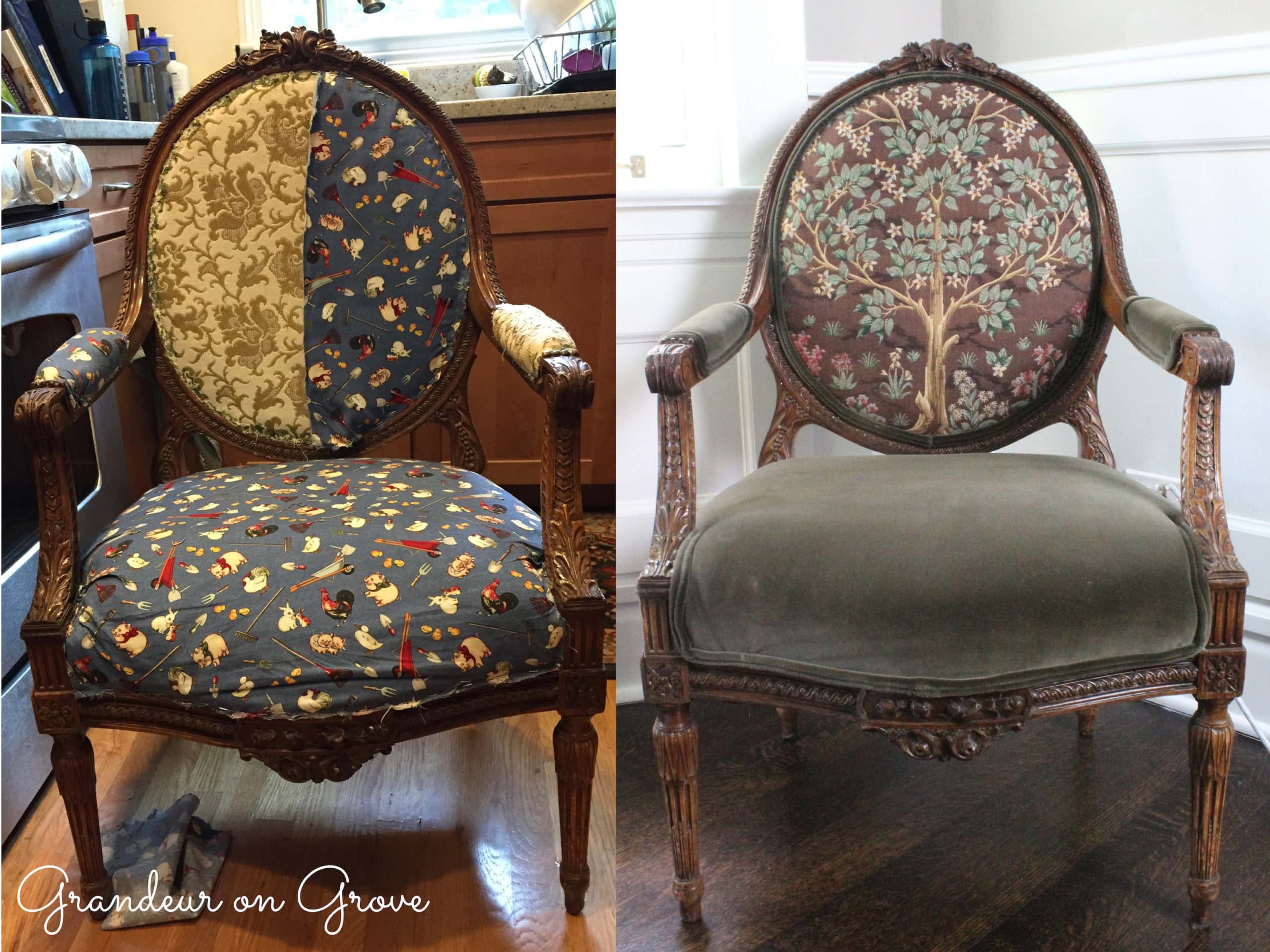This image is a side-by-side comparison of two antique chairs in portrait orientation, creating a before and after effect in a landscape format. Both chairs are ornate and feature oval backs. The chair in the right-hand image is upholstered in greenish gray velveteen with arm coverings in the same color. The backrest is adorned with a detailed picture panel of a tree, featuring gold branches and matching green leaves. This chair sits on a diagonally sloping dark hardwood floor with white walls behind it, showcasing a careful restoration that brightens the frame's lighter wood.

Conversely, the chair on the left retains its antiquated fabric and features mixed upholstery with right-side cushions in navy blue adorned with random patterns, while the left side of the backrest is in a cream fabric with a gold motif. Its ornate legs and armrests are consistent with the right chair but seem less vibrant. This chair is placed against a background featuring room furnishings, such as a silver oven, a counter with a sink, and a dish strainer in the top right corner above brown cabinets.

At the bottom left corner, the white text reads "Grandeur on Grove," indicating the location. This image captures the contrast between a historic and a refreshed appearance, emphasizing the heritage and transformation of these antique pieces.